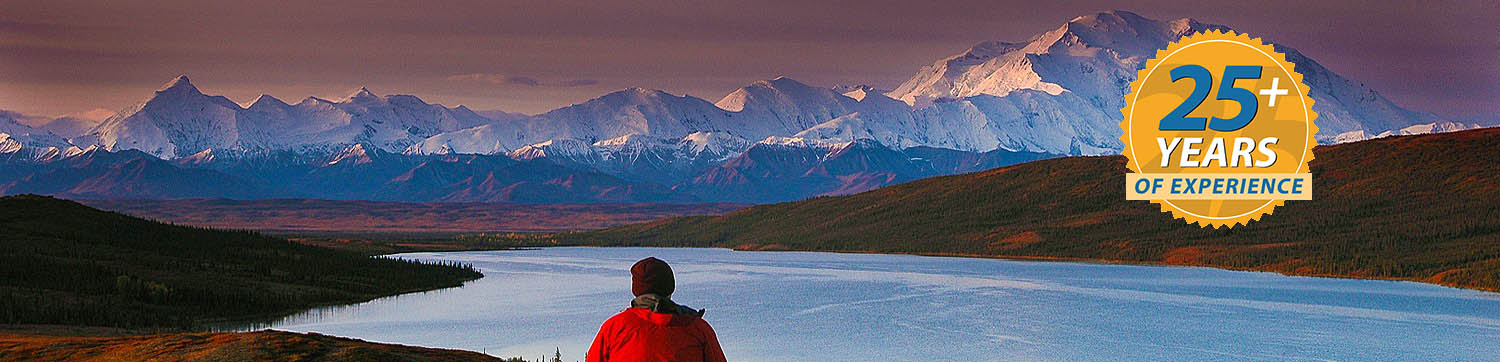In this horizontally oriented image, a person is standing with their back to the camera, wearing a red jacket and a dark red knit cap. The individual is positioned at the base of what appears to be a glacier, facing a frozen body of water, which could be a lake, ocean, or river, surrounded by green and brown land. The scene is set against a long, horizontal mountain range covered in snow, which might be Mount Denali, indicating a location potentially in Alaska. The backdrop features a sky tinged with shades of purple and blue horizontal lines, suggesting late evening with overcast conditions but some sunlight. On the right side of the image, there's a gold seal graphic that reads "25+ years of experience," possibly indicating that the image is from a website or advertisement for a tourist destination or guided tour service.